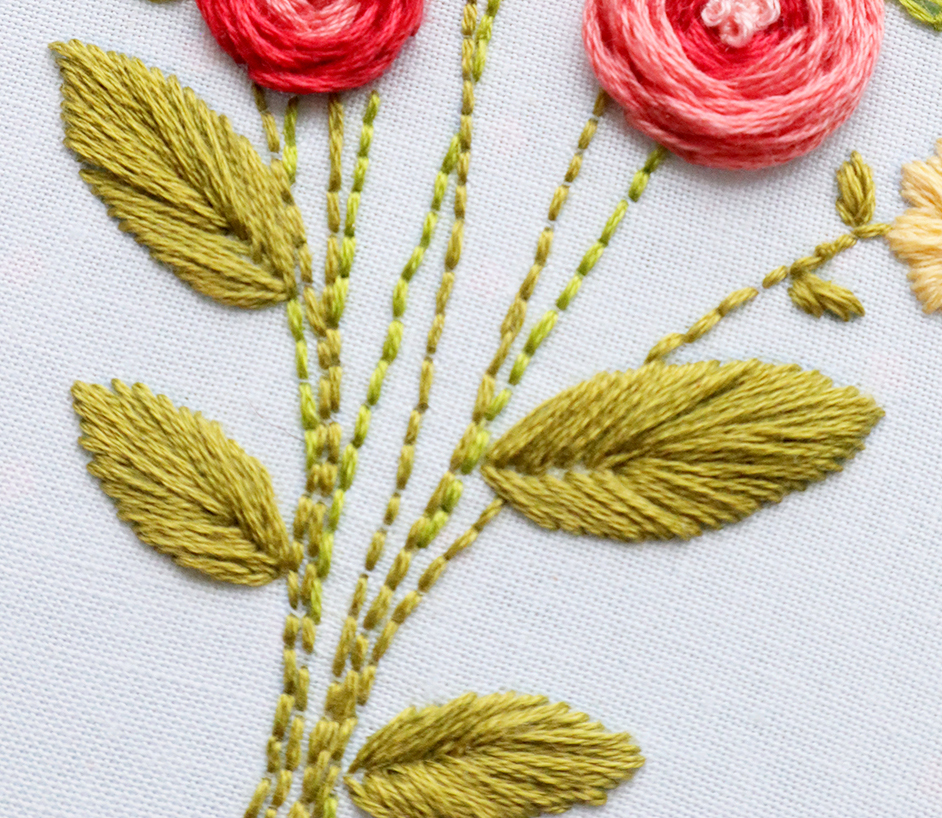This close-up image features an intricately crafted flower design, likely accomplished through cross-stitch or embroidery on a white canvas backdrop. The central focus is on an array of flowers, predominantly pink and red roses with detailed green leaves and stems. Notably, one pink rose has a darker fuchsia outer edge, while another features a deeper fuchsia center with lighter pink on the outside. Adding to the floral ensemble, a glimpse of a yellow flower appears on the right edge of the image. The design also includes delicate, curly pink stitches at the center of the flowers, providing an extra touch of elegance. The stems and leaves in greenish-yellow thread extend upwards, some disappearing beyond the top edge of the photograph, emphasizing the vivid contrast against the clean white background. This image captures the meticulous details and vibrant colors of the embroidered floral art, celebrating the craftsmanship behind it.